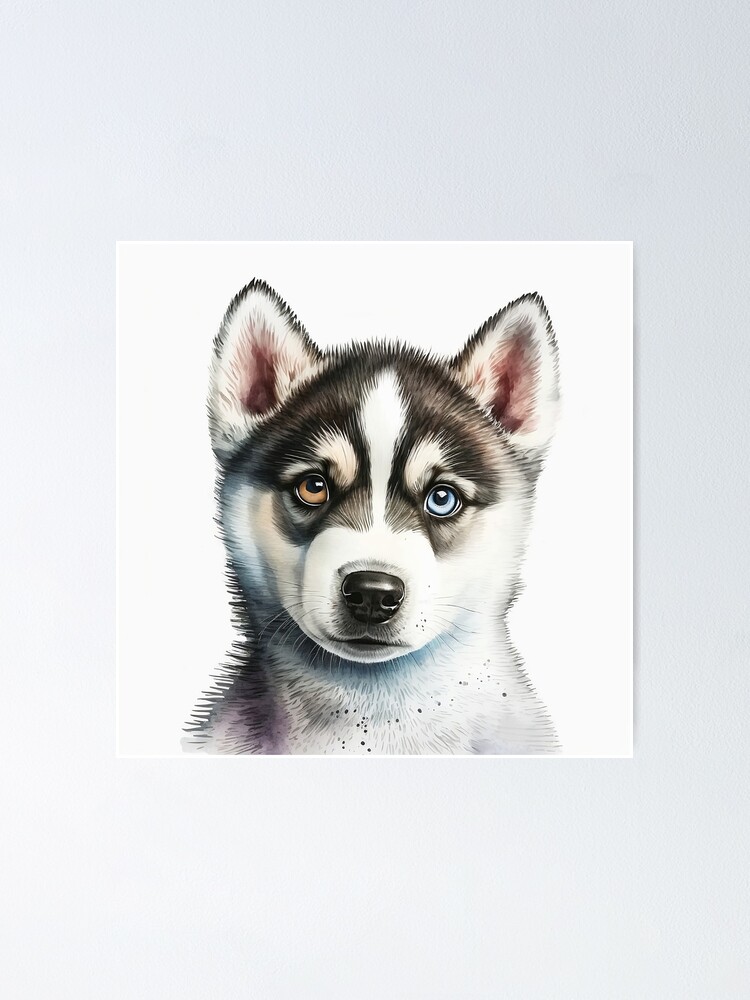This detailed computer-generated artwork features a frontal head and neck portrait of a curious yet calm husky against a white background. Mounted on a light blue mat and distinguished from the slightly grayish-white wall on which it hangs, the husky's vibrant character is brought to life through meticulous strokes. The dog gazes forward with striking heterochromia; its right eye is a piercing blue while its left eye is a warm brown. The husky, with pointed ears lined in faint pink, has striking black and white fur—showcased through a bandit-style black mask, a white stripe down its nose, and subtle gray shading on its upper body. Each black eye mask is highlighted with distinct white markings above, resembling eyebrows, adding to the lifelike quality of this artistic piece.